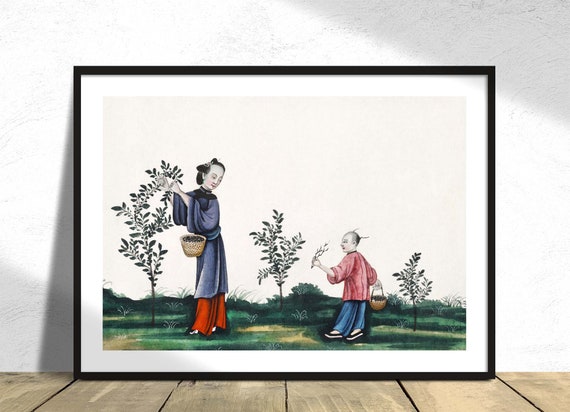The image depicts a detailed painting framed in black, placed on a brown hardwood floor. The painting features two Asian figures amidst a serene, green grassy field with three trees of varying heights—a large tree in front of a woman on the left, a medium tree in the center, and a small tree behind a child on the right. The woman, possibly a geisha, wears a long gray robe with loose sleeves and has purple-red pants beneath. She carries a white basket under her left arm and gazes back at the young boy, who is dressed in a pink shirt, blue pants, and black-and-white sneakers. The boy also holds a basket and appears to be examining flowers or berries he picked from the trees. The backdrop of the scene is entirely white, enhancing the vivid colors and intricate details of the figures and their surroundings. The scene on the painting is bordered by the black frame that rests firmly on several wooden planks, blending the rustic and serene elements harmoniously.